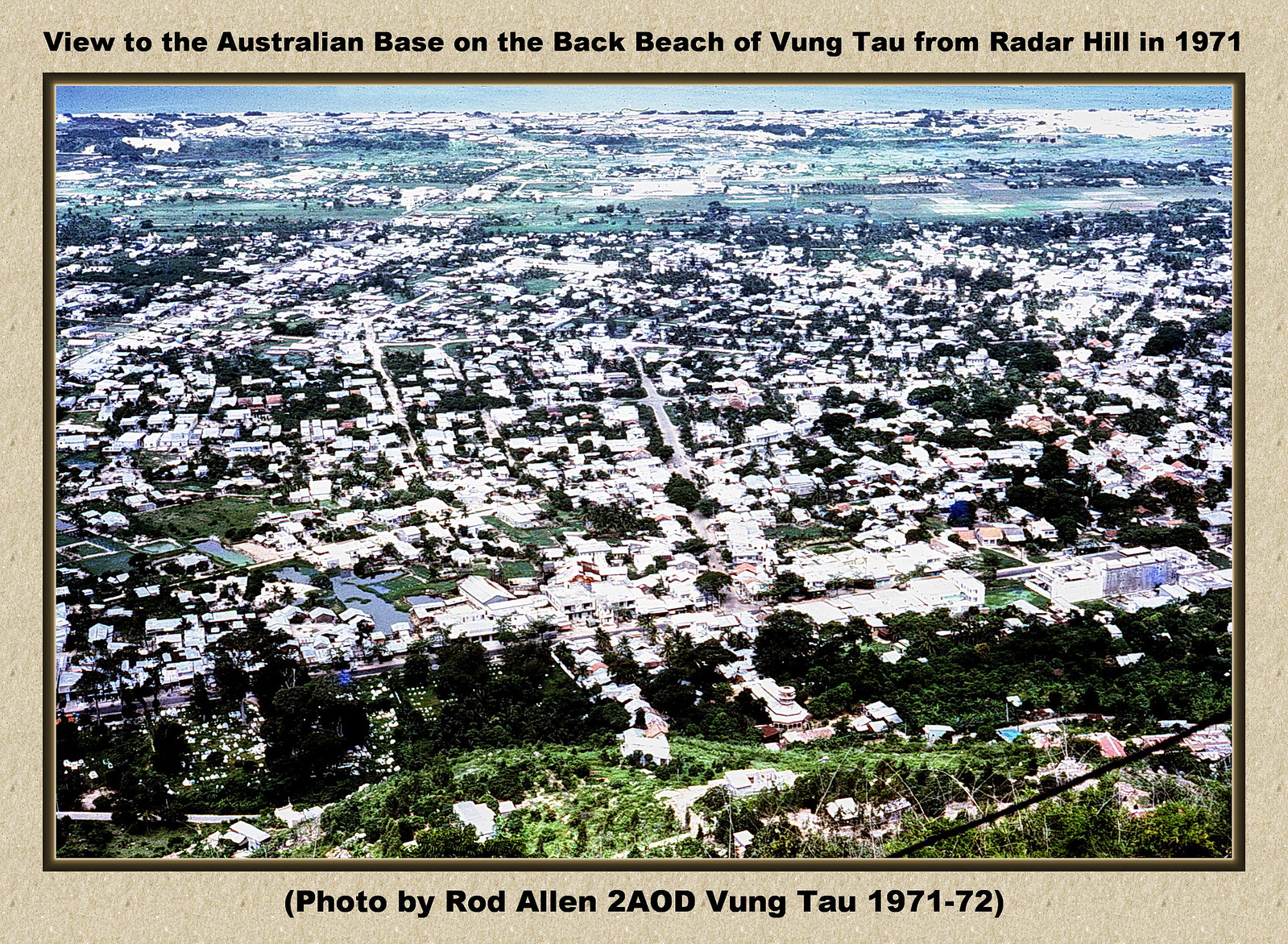The photograph captures a high-elevation view of Vung Tau, taken from Raider Hill in 1971, and conveys the sprawling cityscape below. The urban area, densely packed with houses featuring predominantly white roofs, stretches across the majority of the image. Interspersed among the buildings are patches of greenery and tree-lined streets. In the distant background, a hazy expanse that looks like grassland can be seen. At the bottom right corner, a black diagonal line, likely a telephone or electrical wire, cuts through the scene. The sky forms a narrow, serene blue band at the top of the image. There is black text at the top of the photo reading, "View to the Australian base on the back beach of Vung Tau from Raider Hill in 1971," and at the bottom, in parentheses, "Photo by Rod Allen, 2AOD, Vung Tau, 1971-72."